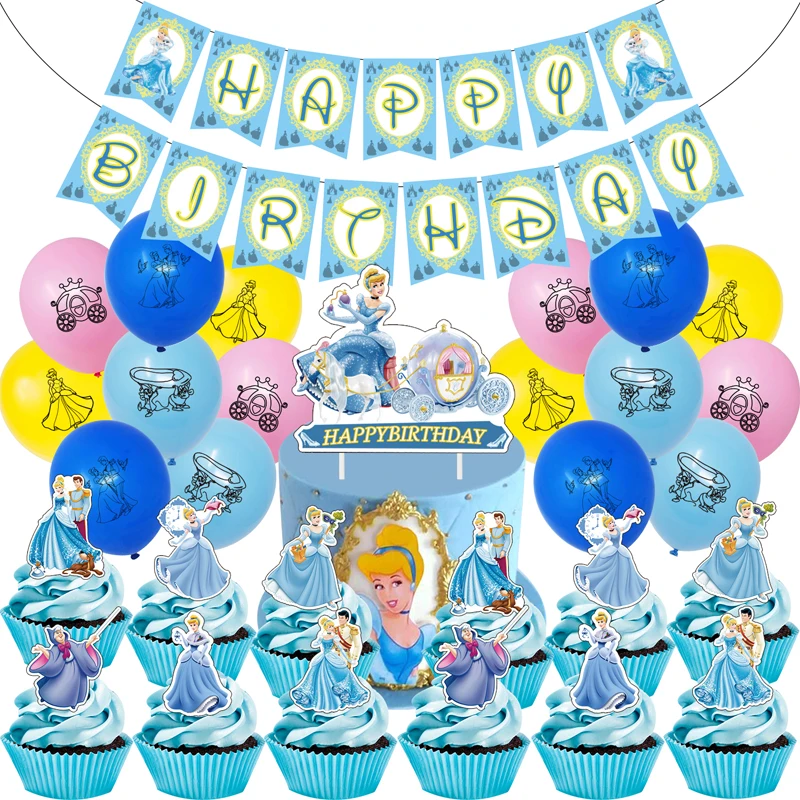This image depicts a colorful, princess-themed birthday scene prominently featuring Disney's Cinderella. At the top, a banner with a "Happy Birthday" message frames the setting, flanked by vibrant balloons of various colors—blue, pink, and yellow. Each balloon showcases whimsical designs: a blue balloon portrays a man and woman dancing in their bed, a yellow balloon features Cinderella alone, and a light blue balloon displays two mice holding a shoe. 

Centrally positioned is a large birthday cake adorned with the same "Happy Birthday" message and an image of Cinderella in a glossy blue dress, holding two purple accessories. Surrounding the cake are numerous cupcakes, each decorated with different characters, including the prince and princess together, Cinderella solo, and the Fairy Godmother. The overall dominant color themes are blue and yellow, with occasional touches of pink, enhancing the festive and magical atmosphere typical of a child's birthday celebration.